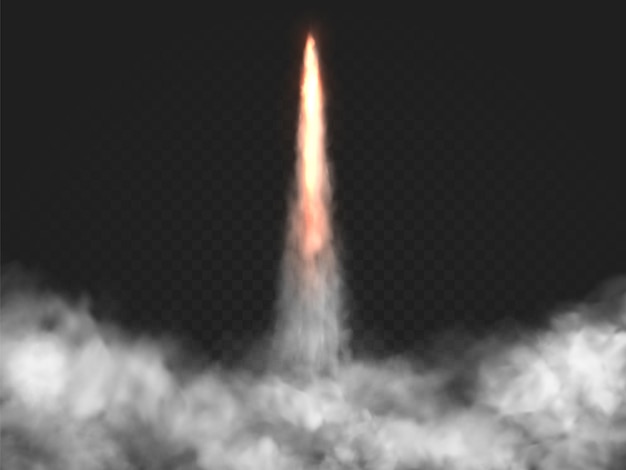The image is a blurry color photograph, possibly computer-generated, depicting what appears to be the jet thrust of a rocket in mid-launch. The rocket itself is not visible, but a line of red fire stretches vertically from the bottom to the top center of the image, fading into black space at the top. At the base of this fiery trail, white smoke billows outward and spreads along the bottom of the image. The background is shrouded in darkness, emphasizing the intense red and white hues. Additionally, a checkerboard watermark pattern overlays the dark portions of the image, contributing to the overall blurred effect.